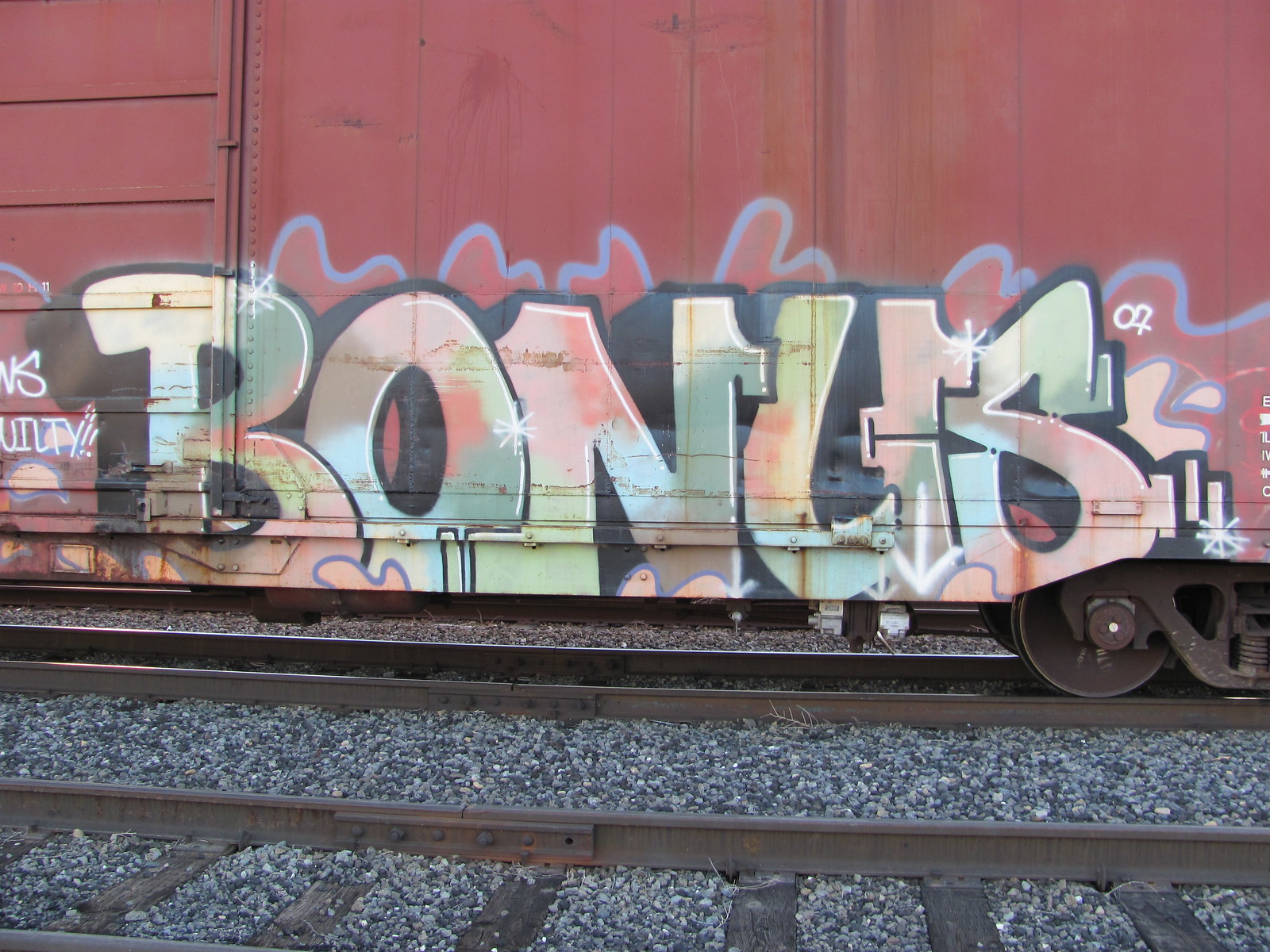The color photo captures a rust-colored train car situated on a set of dark metal and wood train tracks, with stones scattered on the ground between the tracks. One prominent brown metal wheel is visible on the train car. The car itself, rust-colored and aged, features graffiti, with the word "BONUS" in capital letters of various colors—red, blue, and green. The graffiti appears faded, with additional indistinct graffiti visible along the edges of the image. The scene unfolds outdoors in the middle of the day, centered around the railroads and the train standing on them, conveying a gritty, industrial atmosphere.